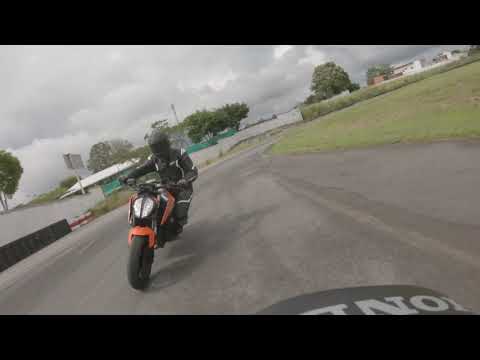The image captures a dynamic scene from what appears to be a rear-facing camera mounted on a motorcycle, filming another motorcyclist behind. The camera is tilted, suggesting the motorcycle is leaning to the left, possibly during a hard turn. Visible on the seat of the motorcycle we are on are the letters "OND," likely part of the word "Honda" in white letters on a black background. The following motorbike is reddish-orange, ridden by a motorcyclist dressed in an all-black suit with a matching black helmet. The rider is leaning far left, emphasizing the tilt while navigating a sharp turn on a grayish-black asphalt road. Surrounding the scene are grassy areas, buildings, and distant trees, under a cloudy sky. The image quality is somewhat grainy and pixelated, adding to the impression that this is a video still.